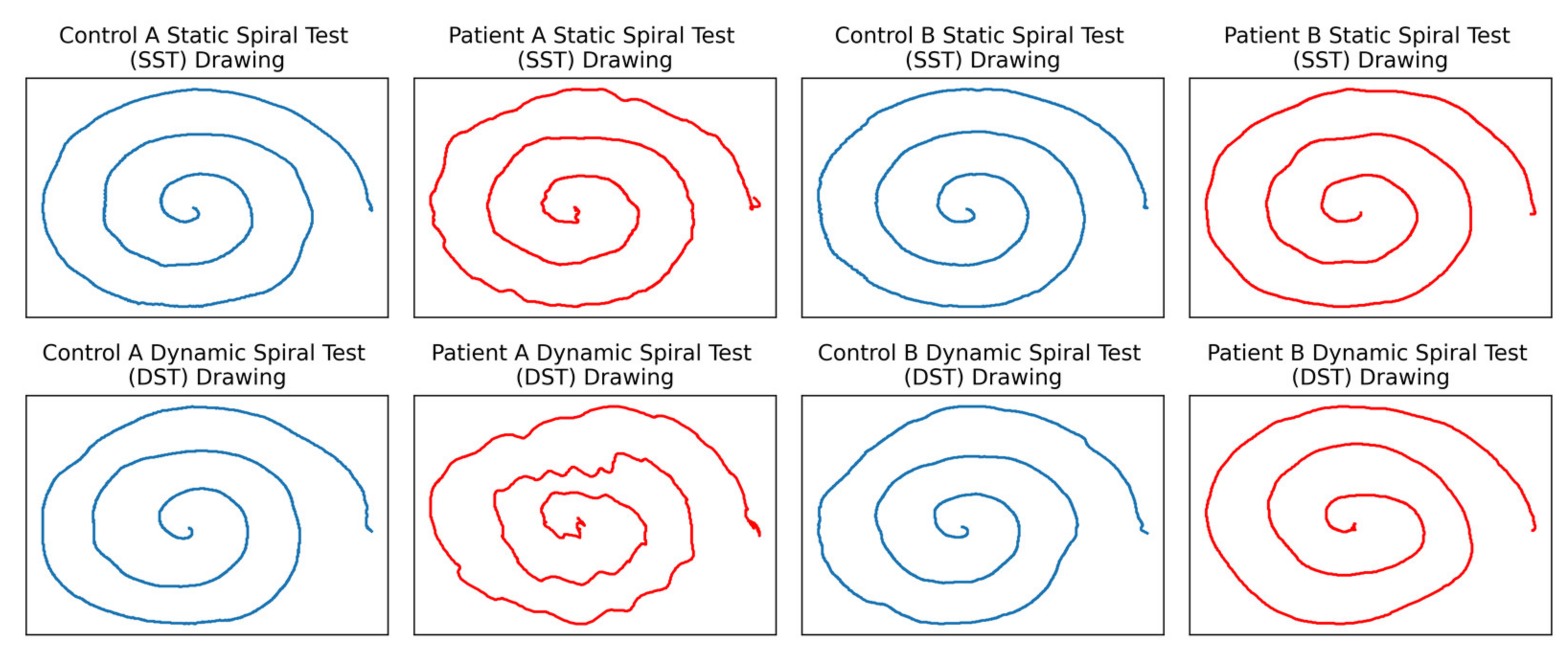The image is a detailed graphic display consisting of eight rectangular panels arranged in four rows and two columns. Each panel contains a spiral drawing rendered in either blue or red ink. The top row captions read "CTRL A Static Spiral Test (SST) drawing," "Patient A Static Spiral Test (SST) drawing," "CTRL B Static Spiral Test (SST) drawing," and "Patient B Static Spiral Test (SST) drawing," respectively. The second row mirrors the top row but alternates with different text indicating dynamic tests, namely "CTRL A Dynamic Spiral Test (DST) drawing," "Patient A Dynamic Spiral Test (DST) drawing," "CTRL B Dynamic Spiral Test (DST) drawing," and "Patient B Dynamic Spiral Test (DST) drawing." 

The panels containing designs drawn by the control group are colored blue in rows 1 and 3, while those by the patient group are red and located in rows 2 and 4. A notable distinction is found between the smooth spirals in most panels and the more jagged, squiggly spirals of the patient drawings in columns 2, particularly in both the static and dynamic tests indicating "Patient A." This variance sheds light on the differing characteristics between the subjects under study, highlighting the contrast in their spiral drawing patterns.